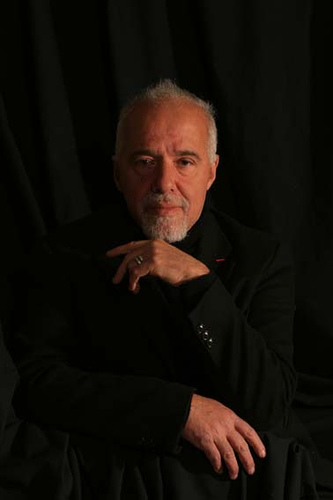In this highly detailed close-up portrait, an older gentleman, possibly in his sixties, is clad entirely in black, including a long-sleeved jacket adorned with three buttons at the cuffs, a black shirt, and black pants. A hint of red can be seen near his lapel. His short-cropped white hair sharply contrasts with his dark eyebrows, and he sports a receding hairline, a neat white goatee, and a mustache. 

The man, who evokes the appearance of well-known figures such as Bruce Springsteen or Tom Jones, has a distinctive silver ring on his left ring finger. His left hand rests beneath his chin in a relaxed gesture, while his right hand lies on his lap or an object draped in black cloth. The backdrop is a loose black curtain, creating a dramatic contrast to the man's pallor and black attire. An asymmetrical lighting from the right casts shadows, adding depth to the photograph. This type of posed and polished image could easily be used for a brochure, a speaking engagement, or an author's profile.